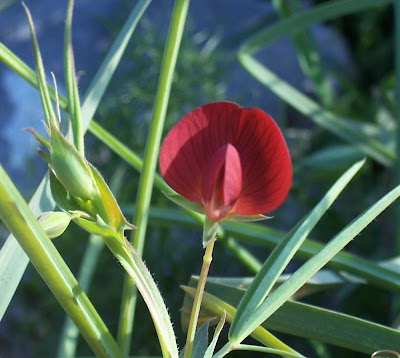This captivating photograph showcases a vivid red flower in full bloom, prominently positioned nearly at the center of the image, slightly skewed to the upper right. The flower features four petals, with two fully opened and the other two still partially closed, exuding a sense of emerging vitality. To the left of the main bloom is another stalk with a green bud, hinting at its imminent blossoming. The surrounding greenery, composed of random long leaves and additional plant stems, fills the scene with varying shades of green, adding to the lushness and depth of the composition. 

The blurred background in gray-blue tones, likely a sky or another indistinct outdoor element, adds a contrasting calmness to the vivid colors of the plants. This backdrop, coupled with the focused sharpness of the red flower, emphasizes the bloom as the focal point. There are no textual elements to distract from the natural beauty captured. A subtle, unidentified ring can be spotted at the bottom right corner, contributing an element of intrigue. This photograph, taken in what appears to be a real-life outdoor setting such as a garden or yard, beautifully balances the dynamic interplay of colors, textures, and natural growth.